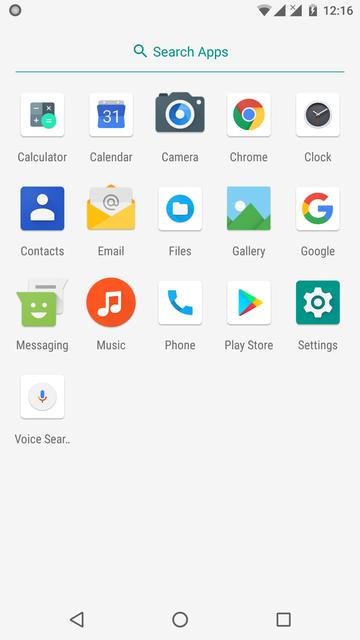The image displays a smartphone home screen set against a gray background with the time shown as 12:16 at the top. Below the time, a search bar with a teal background and a magnifying glass icon is prominently featured, inviting users to search for apps and other content. 

The screen is filled with various app icons arranged neatly in a grid. The visible apps include:

1. Calculator
2. Calendar
3. Camera
4. Chrome
5. Clock
6. Contacts
7. Email
8. Files
9. Gallery
10. Google
11. Messaging
12. Music
13. Phone
14. Play Store
15. Settings
16. Voice Search

At the bottom of the screen, there are three navigation icons: an arrow pointing to the left (back button), a circle (home button), and a square (recent apps button). The "Sear..." text suggests that a search query may have been partially entered.